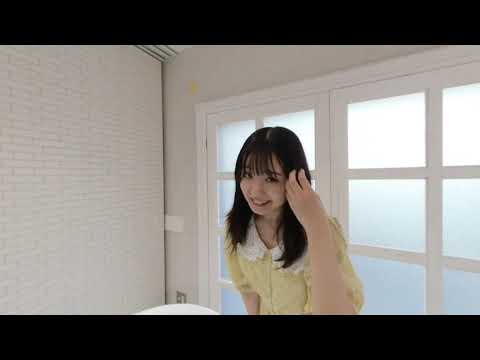The image depicts an Asian woman with long, dark hair, dark eyes, and dark eyebrows, smiling softly while taking a selfie in what appears to be her apartment. She is wearing a light yellow blouse adorned with a white lace collar. The woman is positioned centrally in the photo, leaning slightly forward, with her right arm at her side and her left hand gently combing through her hair. The background reveals a serene indoor setting featuring white walls, a door with white framing, and an opaque set of French doors letting in light, though their glass panes are not transparent. Additionally, there is a small white-brick section to the left, along with a visible light switch. The overall ambiance of the image is calm and relaxed, hinting that it might be intended for a social media profile picture.